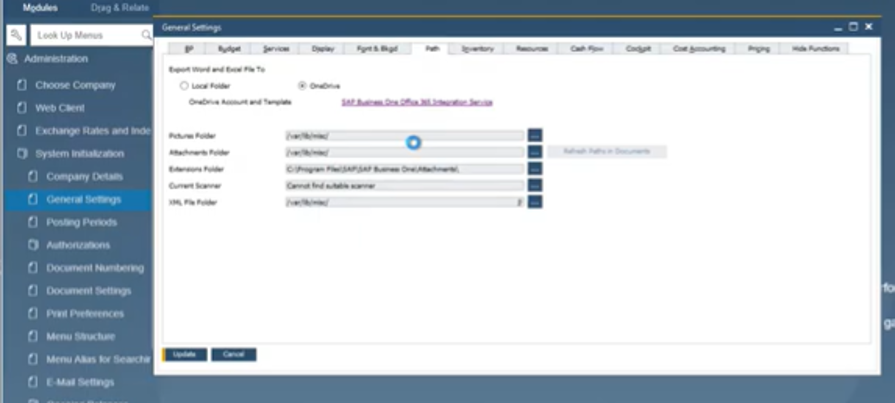The image depicts a blurry and unfamiliar webpage, making it challenging to discern specific details. The available text indicates it's related to "general settings." On the right side, a dark blue section contains headings, with "Choose Category" at the top. The indistinct top heading might offer clues about the webpage's purpose, possibly related to modifying or selecting settings on a computer. Overall, the lack of clarity and context renders the page difficult to navigate or understand, contributing to its tedious nature.